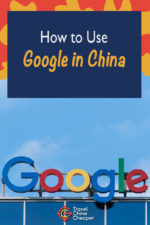This image captures a vibrant design commonly associated with Google's creative branding. The top half of the image features a dynamic background with splashes of red and yellow, suggesting a lively and energetic theme. Foregrounded against this colorful backdrop is a prominent blue box that occupies a significant portion of the image. Inside this blue box, the phrase "How to Use" is displayed in bold white text, with both "How" and "Use" capitalized for emphasis. Directly below this phrase is the word "Google" followed by "in China".

Further down, the visual transitions to a real-world setting, showcasing the top section of a Google office building. Atop this building, the iconic Google sign is clearly visible, indicating its location. The juxtaposition of the vibrant, abstract design with the corporate, real-world element creates an engaging and informative visual experience.